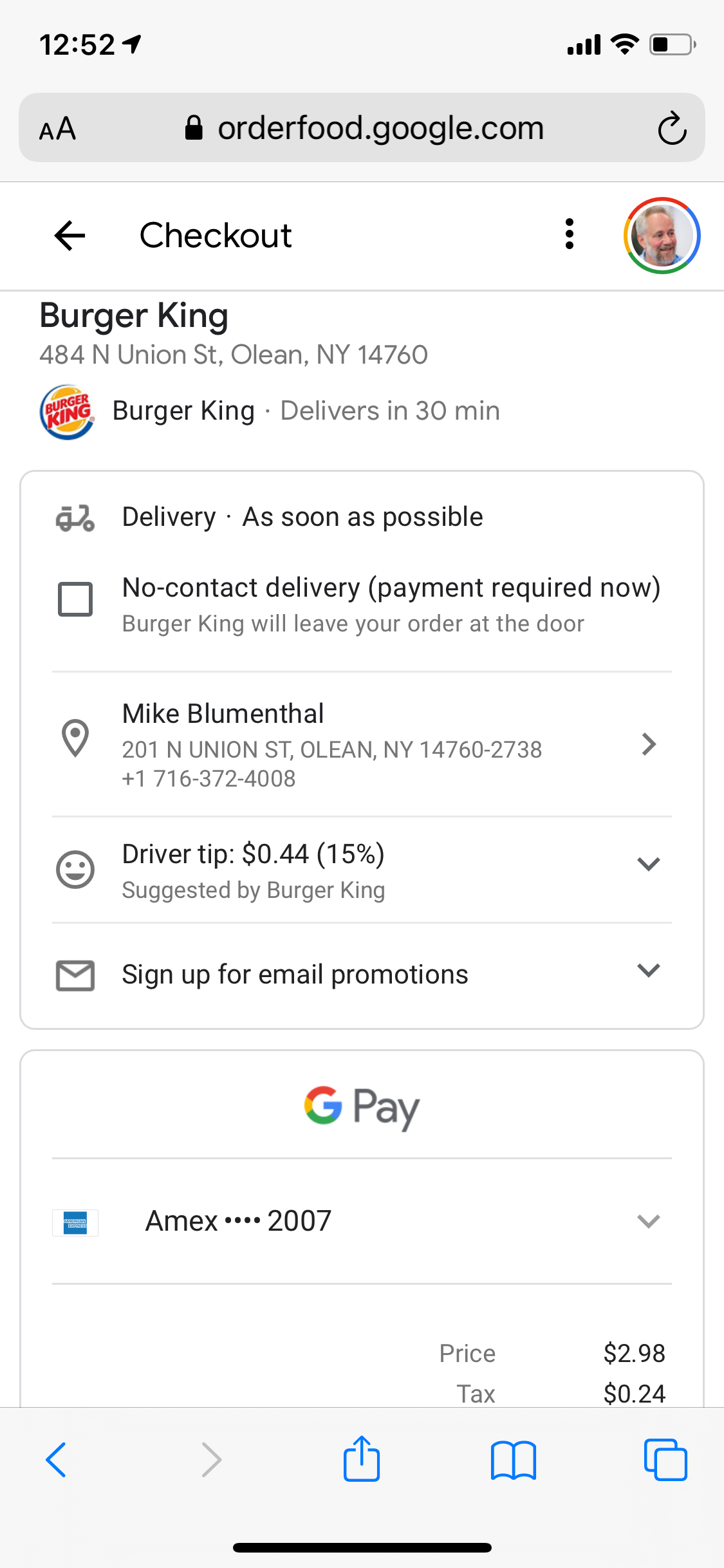This image is a detailed screenshot from a smartphone featuring a food order summary from Google Food Ordering. The background is predominantly white, and the time displayed at the very top left is 12:52 PM, while on the right side, the battery icon indicates the charge level at about one-third. Next to the battery are the Wi-Fi and wireless signal icons, both in black.

Underneath the status bar, the web page URL, `orderfood.google.com`, is displayed against a gray, long rectangular box that stretches from left to right. Below the URL, against a white background, is a black font heading that reads "Checkout," accompanied by a left-pointing black arrow.

On the right side of the heading is a small profile photo of the user, identified as Mike Blumenthal. The photo depicts a white man with gray hair and a salt-and-pepper beard, appearing to be in his late 40s or early 50s.

A detailed section lists the restaurant's name and address: "Burger King, 484 North Union Street, Olean, New York 414760." Similarly, "Burger King" is mentioned again below with information that the delivery will arrive in 30 minutes. Next to this, on the left side, is the iconic Burger King logo, featuring the words "Burger King" in red letters against the background of a hamburger bun.

Below the logo and delivery information, the text "Delivery as soon as possible" appears in dark gray, followed by "No contact delivery (payment required)" indicating that Burger King will leave the order at the door.

Further down, the customer's details are displayed, including the name Mike Blumenthal, his address, and phone number. The driver tip section shows an amount of $0.44, equivalent to 15% of the order, as suggested by Burger King.

Following this, there is an option to "Sign up for email promotions." The bottom section features various payment logos and details, including the Google Payment logo ("G" in Google colors: red, yellow, green, and blue) and the MX logo in blue. The last four digits of the account number are 2007.

Lastly, the total price of the order is highlighted in the lower right-hand corner as $2.98, with an additional tax of $0.24.